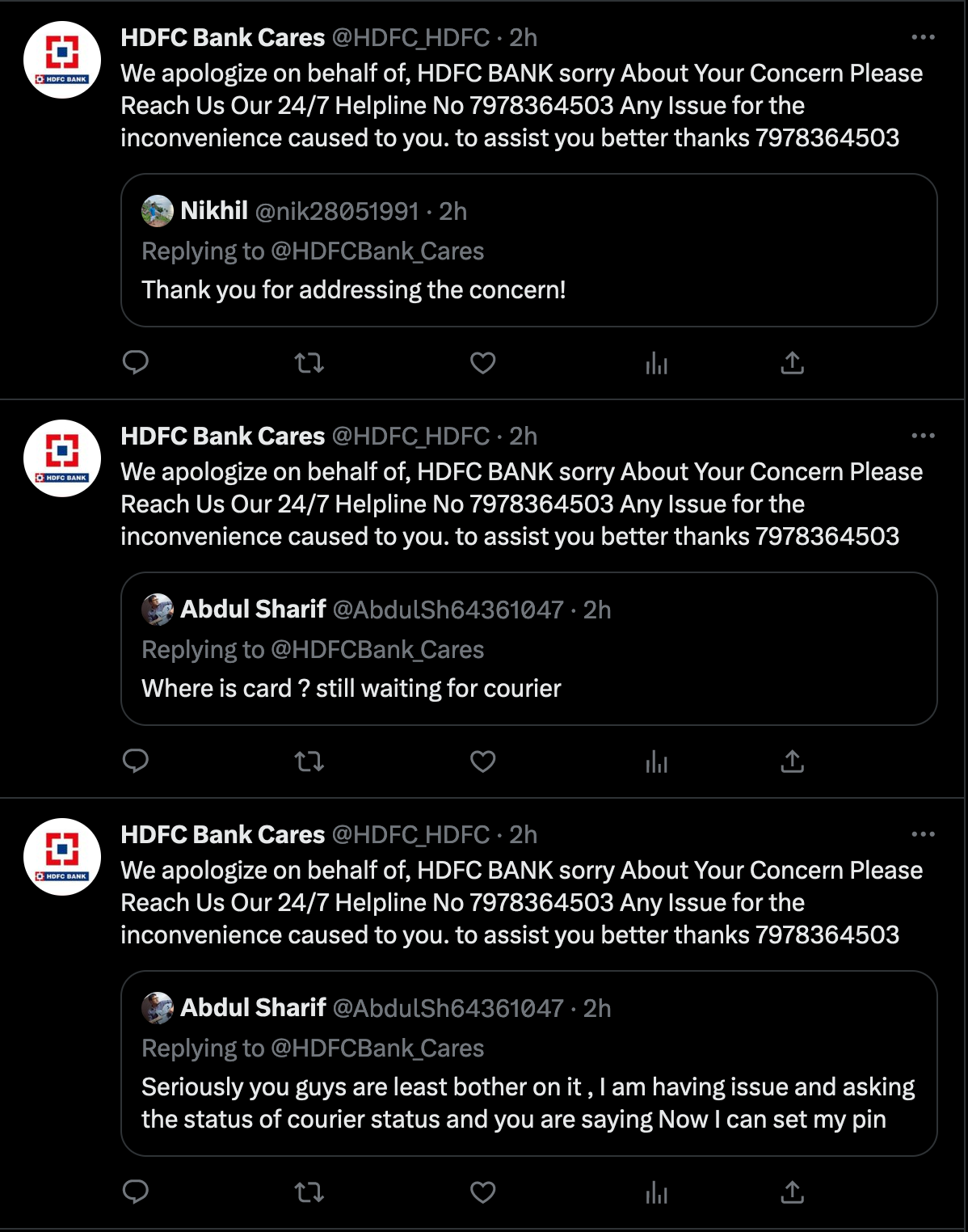The image features a series of tweets prominently displayed. The initial tweet, located at the top left, originates from the account "HDFCBankCares" (@HDFC_HDFC), posted two hours prior to the screenshot being taken. The profile picture for this account is a circle with a white background. Inside this circle sits a square outlined with red brackets, containing a smaller blue square. Beneath these elements within the profile picture is a rectangle with the text "HDFC Bank."

To the right of the profile picture, the username and tweet information are presented. The tweet from HDFC Bank reads: "We apologize on behalf of HDFC Bank. Sorry about your concern. Please reach our 24/7 helpline number at 797-836-4503. Any issues for the inconvenience caused to you to assist you better? Thanks."

Below this tweet, user "Nick Hill" expresses their gratitude with the reply, "Thank you for addressing the concern." Beneath Nick Hill's reply, a row of icons is visible, including a comment icon, retweet icon, heart icon, graph icon, and share icon.

Further down, the same assistance message from HDFC Bank appears, followed by additional user comments. One user asks, "Where is card still waiting for query?" indicating an unresolved issue.